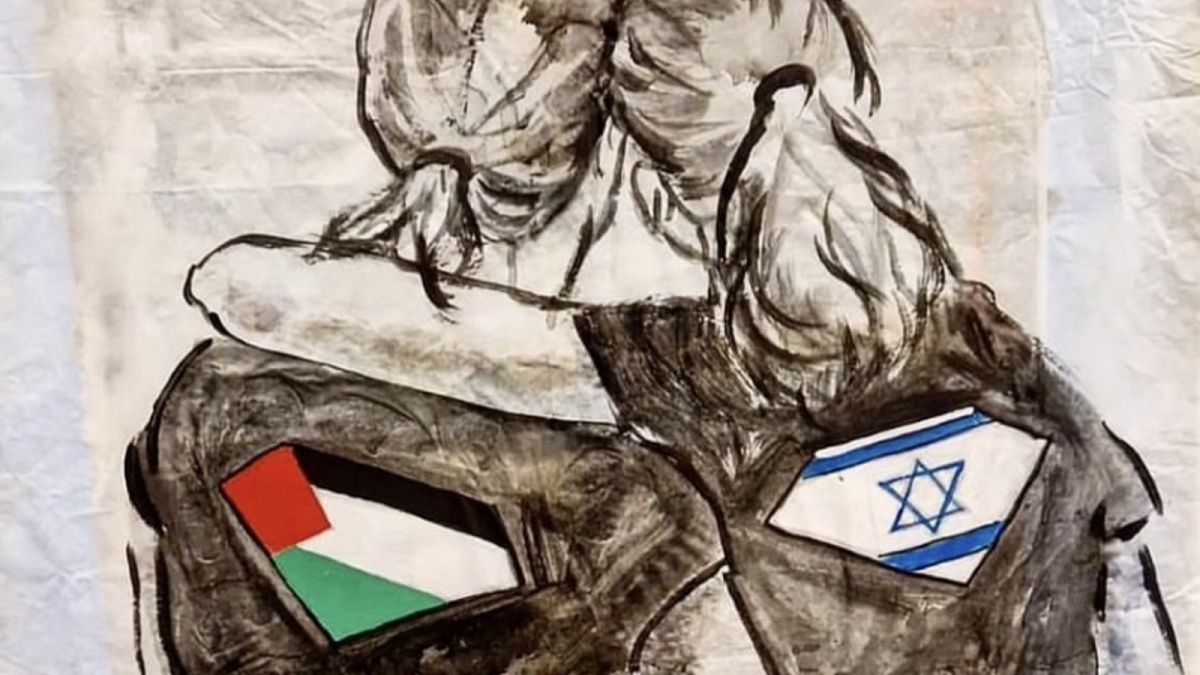This detailed, hand-drawn charcoal or dark black pencil sketch, possibly also using pastel, features two figures, likely women, viewed from the back. Both have long hair tied in ponytails and are wearing black short-sleeved shirts. The figure on the left is adorned with the red, white, black, and green flag of Palestine, while the figure on the right bears the blue, white, and black flag of Israel, identifiable by the six-pointed star. The woman on the right has draped her left arm affectionately around the shoulder of the woman on the left, creating an intimate gesture of solidarity. They stand before a textured, crinkled backdrop devoid of any writing, adding to the raw, emotive quality of the drawing. This artwork, showcasing the embrace, seems to symbolize a hopeful plea for peace and unity between the two nations.